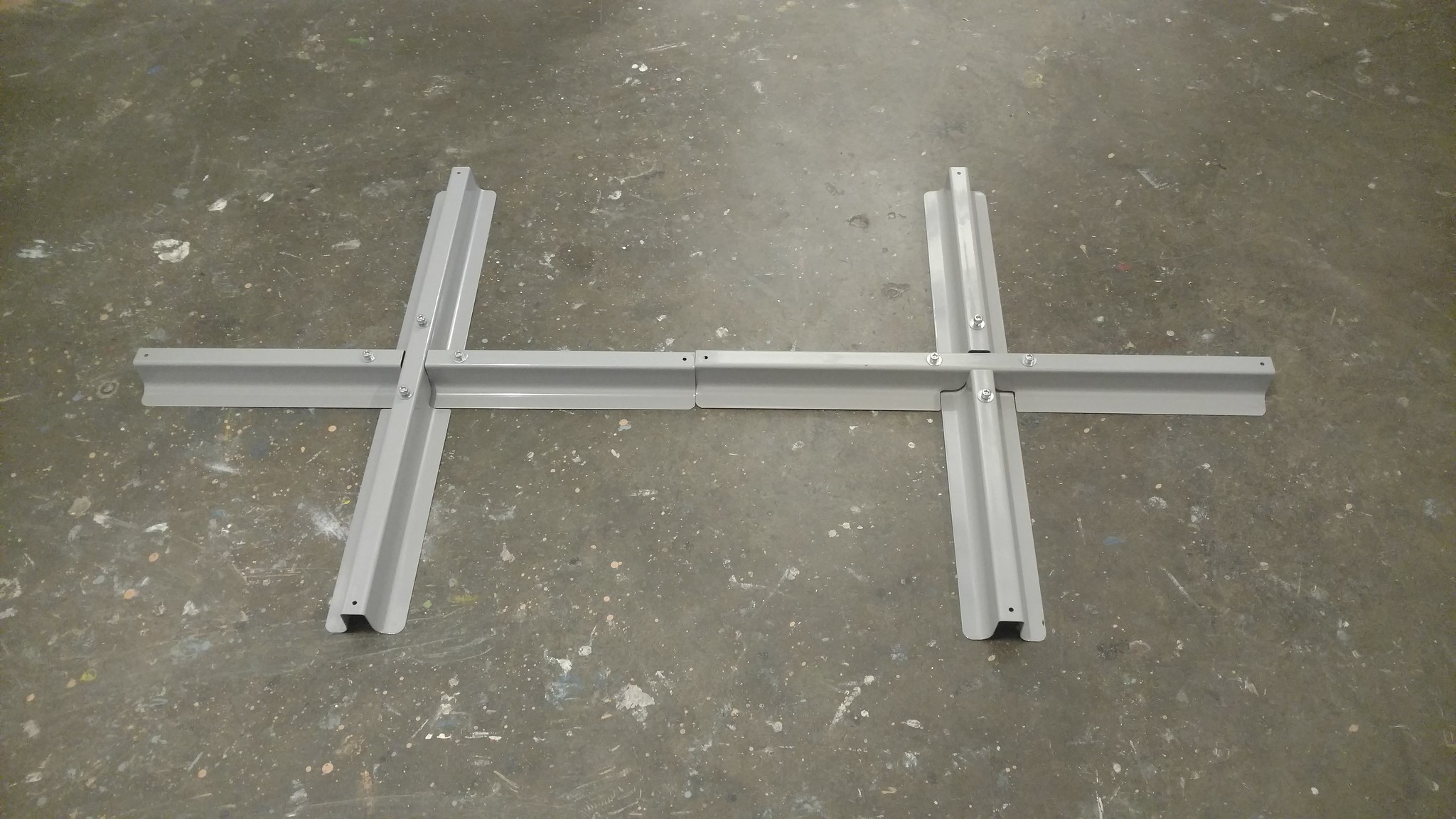The image shows a slightly overhead, angled view of a gray asphalt pavement, which is somewhat smooth but scattered with chips, cracks, and white-colored wear spots. The focal point is a series of six interconnected metal pieces creating a grid-like structure. These metal pieces are light gray or silvery in color and seem to form two sets of plus-shaped assemblies. 

One assembly has a longer central piece, bolted vertically, with shorter pieces coming in from the left and right, forming plus signs. The other assembly mirrors this layout but with the central longer piece positioned horizontally. All metal pieces have hollow channels, suggesting they might be components for a base of furniture, stand, or cable raceways designed to hide and protect cables. These channels are flat on one side, raise up slightly in the middle, and go flat again, characteristic of what is known as a "hack channel". The metal frames appear securely bolted to the pavement, conveying a strong and permanent installation.